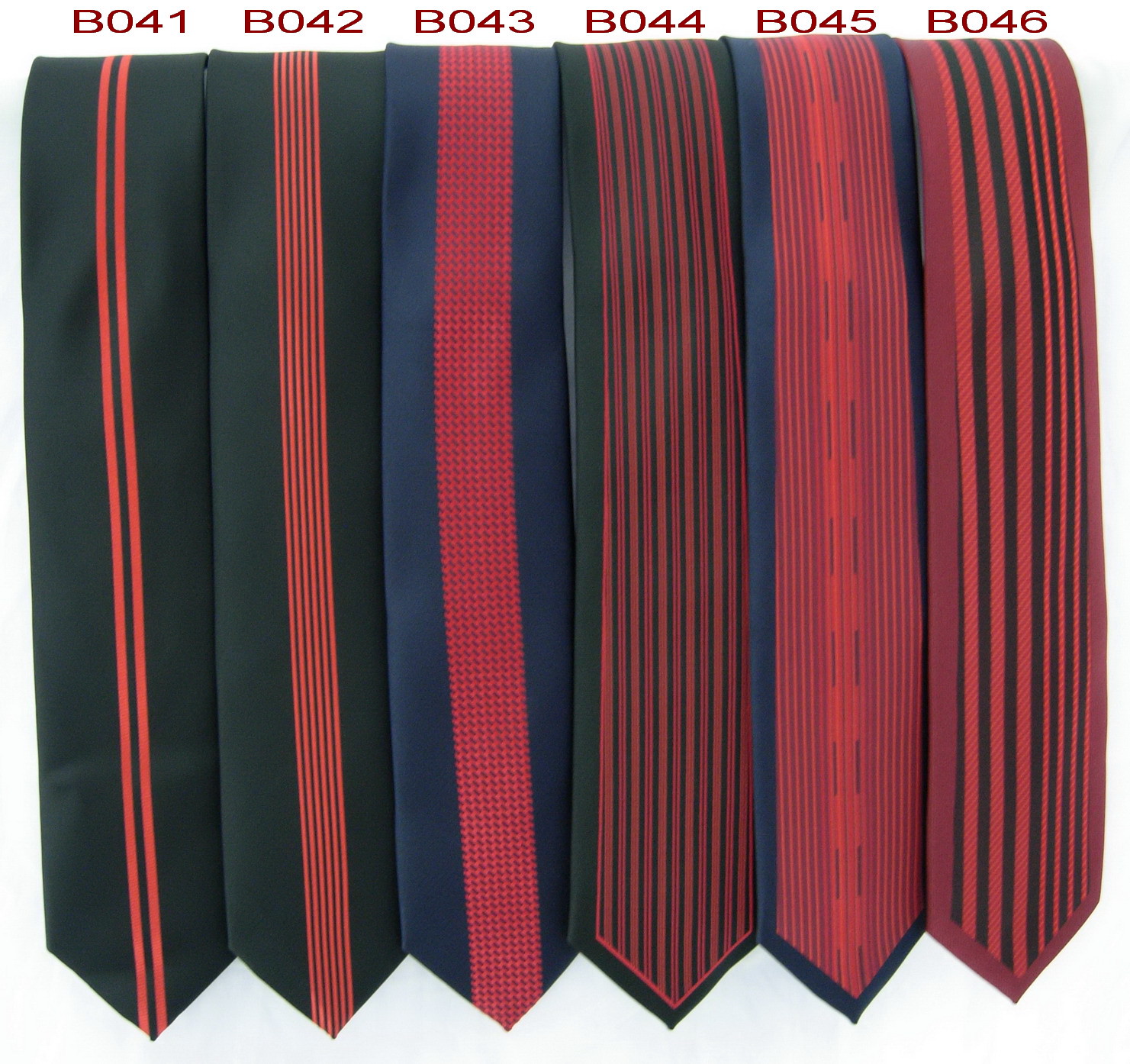This photograph showcases six neckties, possibly from a catalogue, each labelled with maroon numbers at the top: B041, B042, B043, B044, B045, and B046. The ties are displayed in a row, with the pointed ends visible, giving them a distinct tie-like appearance. 

Starting from the left:
- The first tie (B041) is black, adorned with two thin red vertical stripes running from top to bottom.
- The second tie (B042) is a slightly lighter shade of dark grey or maybe even a dark green, featuring six or seven narrow red stripes running vertically.
- The third tie (B043) is a rich midnight blue, characterized by a prominent wide band of textured red stripes, creating a checked effect.
- The fourth tie (B044) appears to be black, with a mix of broad and narrow red vertical lines and black spaces in between, creating a pattern.
- The fifth tie (B045) is predominantly navy blue, with dense red vertical stripes and larger red square block details in the center.
- The last tie (B046) is primarily red, with bold black vertical lines on the left side of the point and smaller, uniform black and red lines on the right side.

Each tie features a unique pattern and color combination, making the collection visually intriguing and varied.